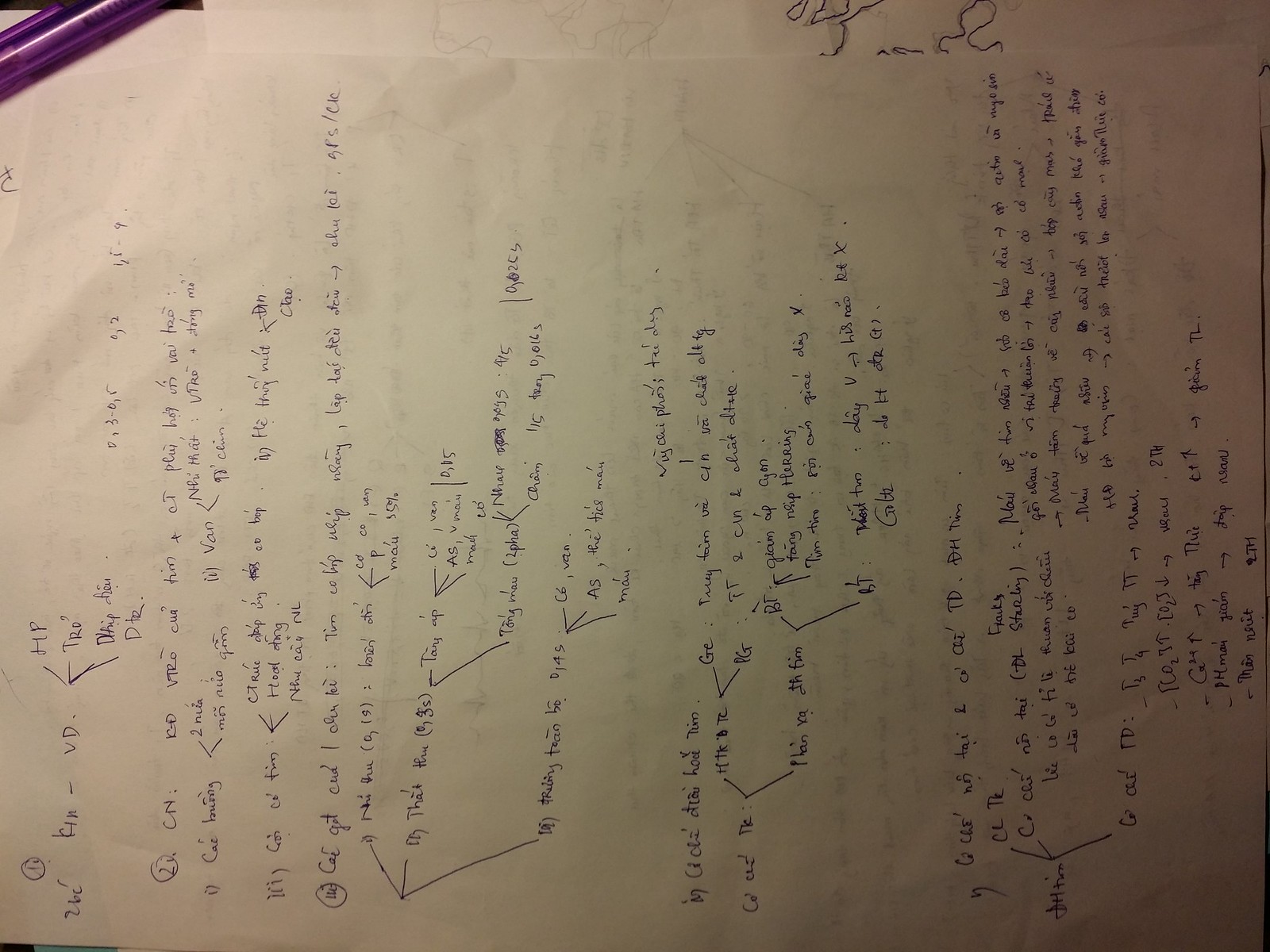This image features a heavily crinkled piece of paper densely covered in text written in very small print. The paper appears to have writing on both sides, with the ink from the reverse side bleeding through, creating an overlay effect. The front side text is primarily written in purple ink, initially appearing to be in English. However, upon closer inspection, the text transitions into what seems to be another language, possibly French, though this is not certain.

The writing is meticulously detailed, with numerous sections circled and labeled, including at least the numbers one, two, and possibly three. Additionally, the paper is adorned with diagrams that utilize large arrows with lines through the middle, indicating connections or groupings of related items. One of these sections includes an arrow pointing to three written items, followed by additional arrows, forming a complex, interconnected structure. Despite the detailed notation, the foreign language makes the content challenging to decipher.